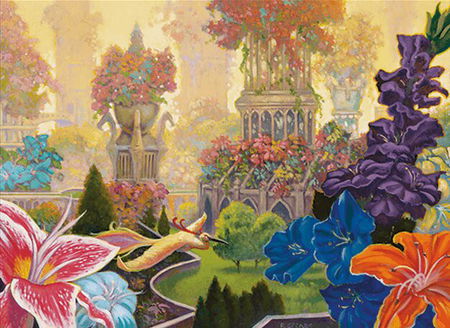The image depicts a vibrant and intricate painting of an elaborate flower garden with a mix of fantastical and realistic elements. Dominating the scene is a circular grass field in the middle, surrounded by various flora and architectural structures. At the center stands a multi-level gazebo-like structure with arched doorways and windows, adorned with a plethora of colorful flowers ranging from yellow and red to blue and pink at its top. To the right of this gazebo, a large vase with swan head details overflows with purple and pink blooms. The bottom right corner showcases an orange flower with adjacent blue and purple plants, while the lower left highlights a mix of red, blue, and white flowers—some resembling lilies with yellow centers. A whimsical element is introduced with a small white figure holding a rake, enhancing the garden's enchanted feel. Various statues and columns with flowers extend throughout the left and upper portions of the image, contributing to the garden's lush, almost magical atmosphere. To complete the scene, a vibrant yellow bird with red head feathers and a long black beak is perched prominently, resembling a peacock, which adds a lively, exotic touch to this garden masterpiece.